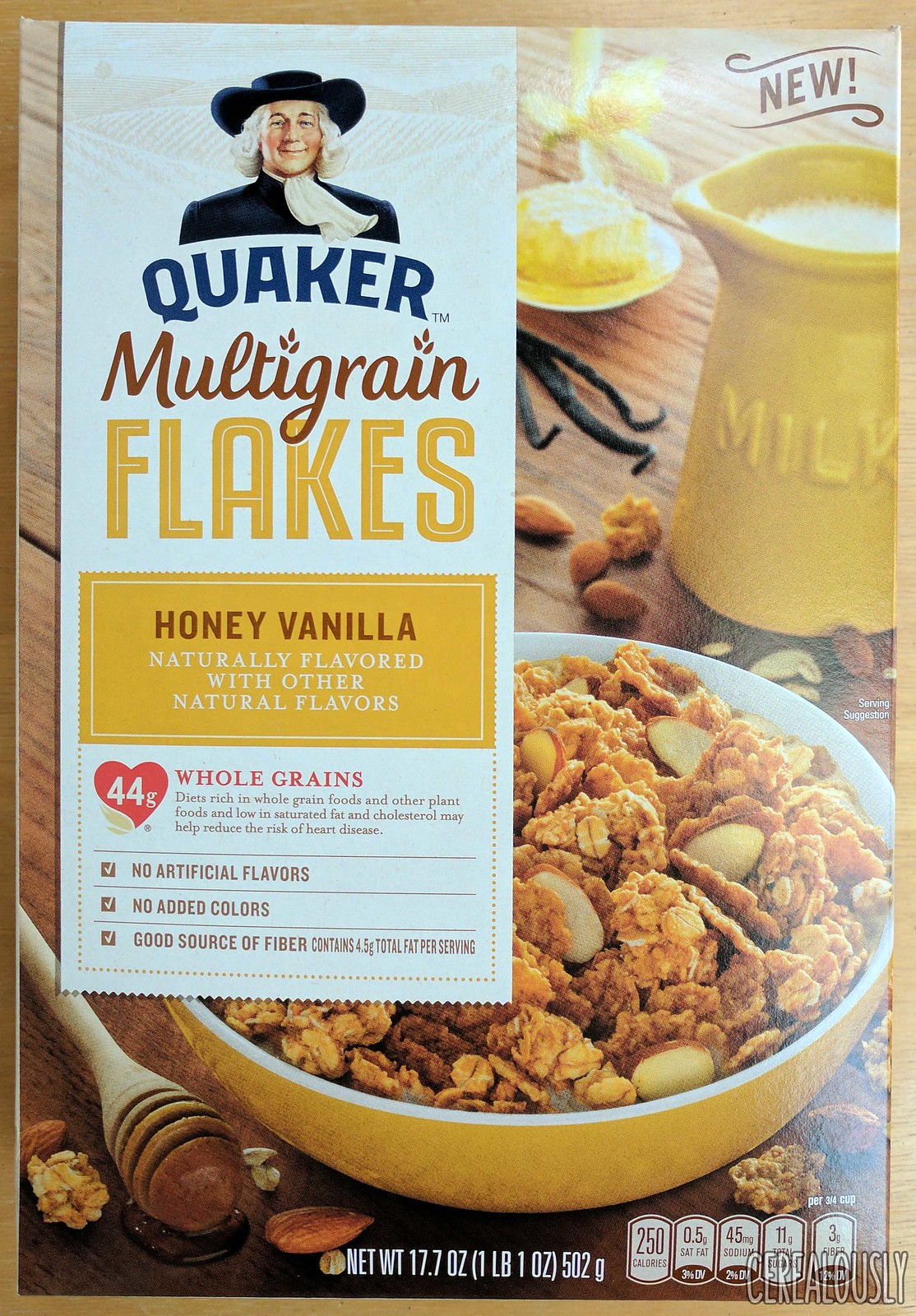This image depicts the front of a Quaker brand cereal box. Prominently displayed at the top is the iconic Quaker logo, featuring the cheerful Quaker man adorned in a black hat, black shirt, and white neckerchief, with his characteristic rosy cheeks and white hair. Beneath the logo, the cereal's name, "Multi-Grain Flakes," is boldly displayed, with "Honey Vanilla" indicating the flavor.

On the left-hand side of the box, a detailed label informs consumers of the cereal's nutritional benefits: "44 grams of whole grains," "No artificial flavors," "No added colors," and "Good source of fiber."

Behind this informative label is a vibrant image of the cereal itself, presented in a yellow bowl. The bowl showcases a mix of crunchy flakes and nuts, bringing the cereal to life. Above this, a yellow carton labeled "milk" is pouring into the bowl, making the scene even more appetizing.

The entire arrangement is set against a rustic wooden table, adorned with assorted breakfast items, including a honey dipper, adding to the cozy, homey feel of the image.